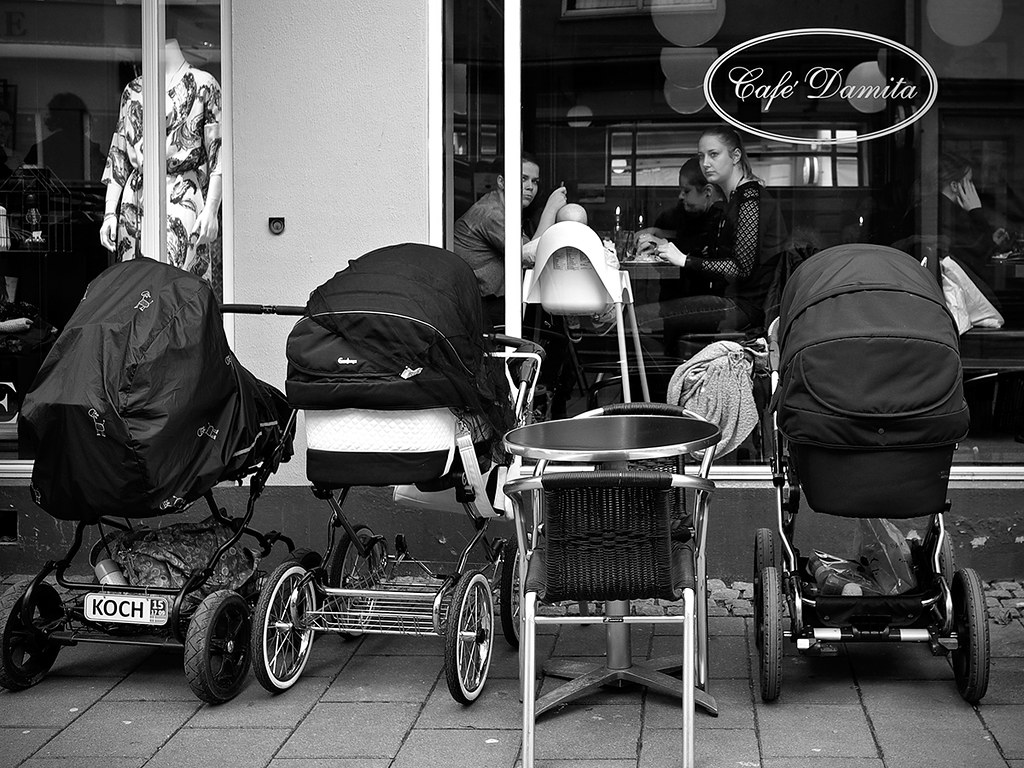This detailed black-and-white photograph depicts an outdoor scene in front of Cafe Damita. Through the large square window of the cafe, three women are visible, with one of them attending to a baby in a high chair. All three women appear to be gazing outside. In front of the cafe, lined up against the wall, stand three baby strollers—one of which is marked with the brand name "Kosh." An outdoor seating area featuring a wicker chair is unoccupied. To the left of Cafe Damita, a retail store with a headless mannequin dressed in a silk robe is partly visible, separated by a stucco divider. The ground outside consists of cobblestones and bricks. The cafe's name is prominently displayed on the window, ensuring the identity of the location.